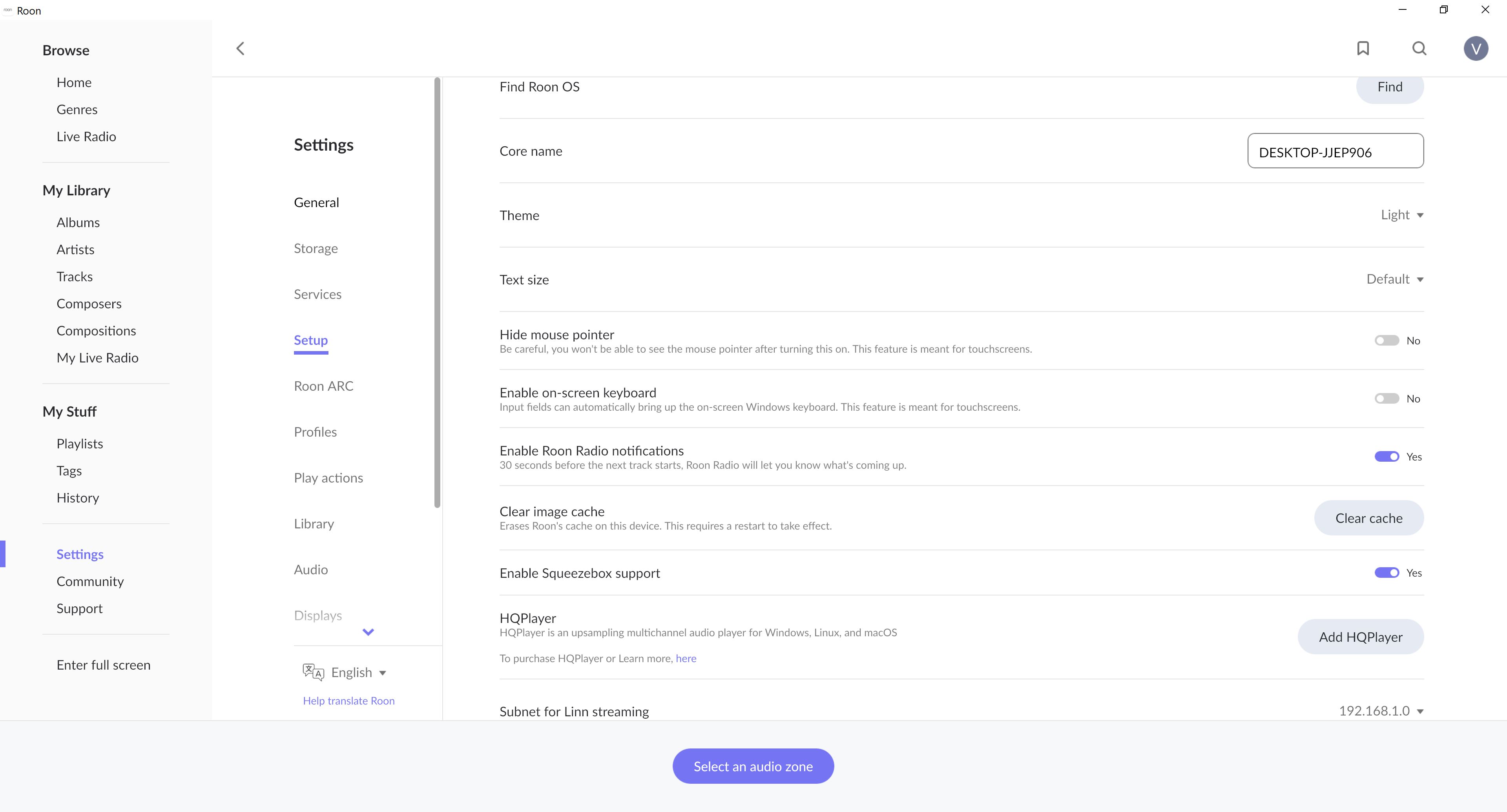**Caption:**

Screenshot: Roon Application Interface

The screenshot displays the interface of the Roon application. At the top right-hand corner, the word "Roon" is prominently displayed. Directly below that, there is a left-pointing arrow next to the word "Browse." Following in a vertical sequence are the options "Home," "Genres," "Live Radio," and "Settings."

On the left sidebar, the categories listed are "My Library" with subcategories such as "Albums," "Artists," "Tracks," "Composers," "Compositions," "My Live Radio," "My Stuff," "Playlists," "Tags," "History," "Settings," "Community," "Support," and "Enter Full Screen."

To the right, under "Settings," there are various configurations listed: "General," "Storage," "Services," "Setup," "Roon ARC," "Profiles," "Play Actions," "Library," "Audio," and "Displays." There's also a language setting, shown as "English" with a dropdown option to help translate Roon.

Further to the right, it mentions "Find Roon OS," followed by settings for "Core Name," "Theme," "Text Size," options to "Hide Mouse Pointer," "Enable On-Screen Keyboard," "Enable Roon Radio Notifications," "Clear Cache," "Image Cache," "Enable Squeezebox Support," "HQ Player," and "Subnet for Linn Streaming." 

A prominent blue button reads "Select an Audio Zone." At the very top right are icons for bookmarks, search, and a user profile depicted by a "V" in a gray square.

Below this interface toolbar, there's a "Find" prompt with an entry box containing "desktop-jjep906." Additional dropdowns and buttons for various settings include options for "Light," "Default," toggles for "No," "Yes," "Clear Cache," "Add HQ Player," and a dropdown for "192.168.1.0."

This detailed interface provides a comprehensive look at the Roon application's settings and customization options.